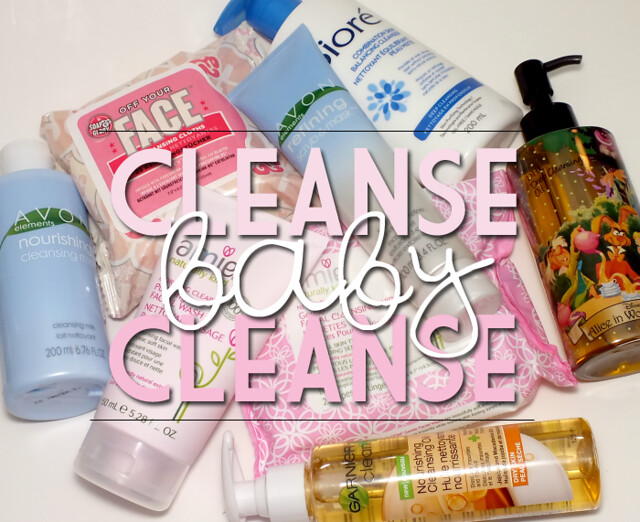This image features a collection of women's beauty and hygiene products meticulously arranged against a clean, white background. Dominating the foreground is bold text that reads "Cleanse Baby Cleanse," with "cleanse" in pink, "baby" in white script, and "cleanse" again in pink. Behind this vibrant text, an assortment of products is displayed, including an AVO nourishing cleanser in a blue bottle with a white cap, an “Off Your Face” beauty cleansing cloth in a pink-labeled square packaging, an Avon refining mask in a blue tube, a Garnier cleanser with an orange bottle and white pump, another cleanser with an orange bottle and distinctive black pump featuring colorful, cartoony designs, and a Biore cleanser in a white bottle with a blue pump. Scattered among these are white tubes suggesting various beauty or moisturizing products, adding to the clean and organized aesthetic of the scene.